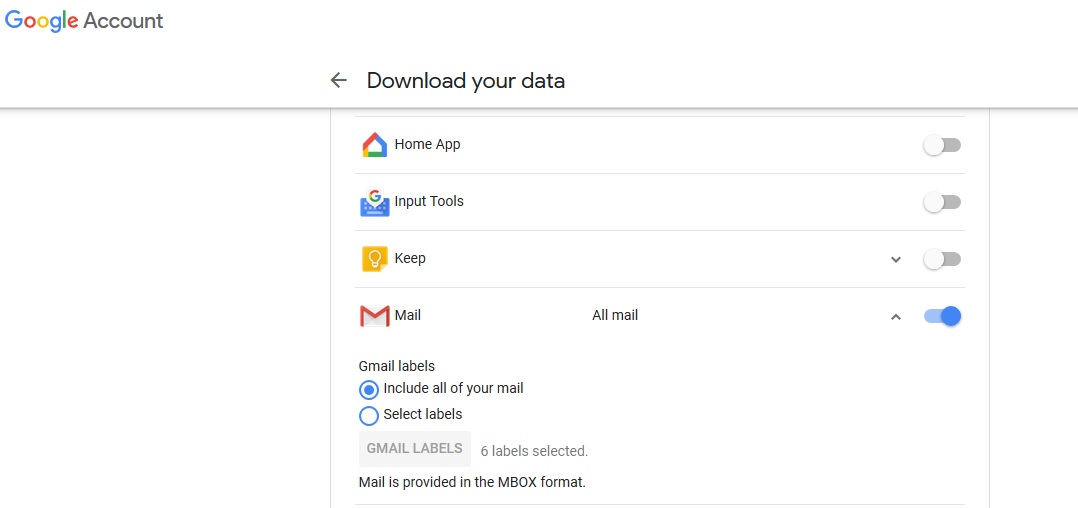Screenshot of Account Settings: Google Account - Download Your Data

The screenshot captures the account settings section of a Google Account, focusing on the 'Download Your Data' feature. At the top left, "Google Account" is prominently displayed, underscoring the user's profile area. Below, the section title reads "Download Your Data," indicating options available for data management.

The first display option is "Home app," which is visibly turned off, followed by "Input tools," also turned off. Next, "Keep" is shown to be deactivated as well. The setting for "Mail (Gmail)" stands out among the options, as it is turned on. Under 'Mail', the user has selected “All Mail,” with the description “Gmail labels on the left include all of your mail," which is confirmed by a blue-filled circle next to it. Another option, "Select labels," is visible but not chosen, as indicated by an empty circle.